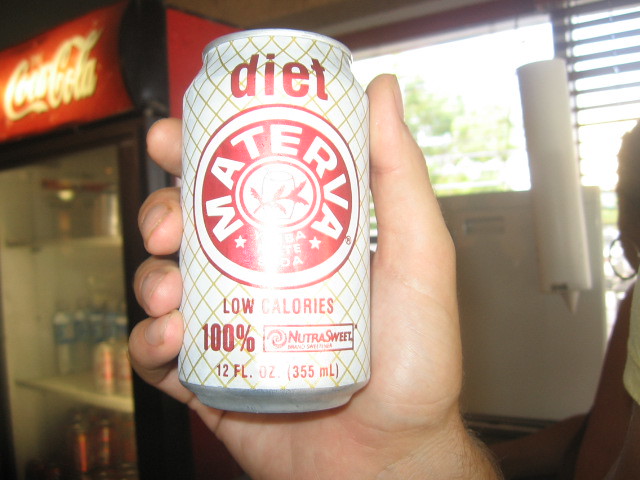In this image, a Caucasian individual's right hand is prominently featured, holding a distinctive soda can. The can is white with a pattern of gold stripes creating an illusion of small white boxes. At the top is the word "Diet" in red text, and the center of the can is marked by an eye-catching red circle. Within this colored circle, the brand name "MATERVA" is inscribed. Due to glare from a light source, some additional text below the brand name is partially obscured. Lower on the can, the phrases "Low Calories" and "100%" are printed in bold red letters, followed by a NutraSweet logo box, and the measurement "12 FL OZ (355 mL)" in red.

The background reveals further elements that help set the scene. There's a window at the back, fitted with horizontal blinds on the right side. In front of the window, a white water dispenser with a cup holder, containing small white cups, is visible. To the left of the hand holding the soda can, there is a Coca-Cola branded cooler, illuminated and filled with various beverages, including water bottles and soda cans. Though slightly muted, the image suggests the presence of another individual off to the right, adding a subtle hint of human activity within the scene.